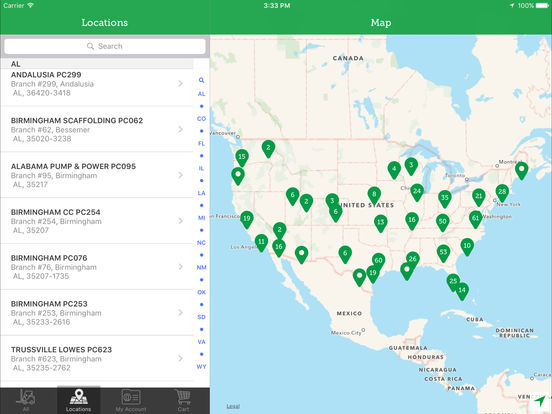This image is a cropped screenshot of a product locator page on a website, featuring a green header at the top. On the left side of the header, the word "locations" is displayed in small white font, while to the right of that, "map" is also in small white font.

Beneath the header, the website interface is divided into two main sections. On the left side, there's an alphabetically arranged vertical list of locations. Each state is separated by a gray box, which includes the state's name followed by its abbreviation (e.g., "Alabama" followed by "AL") and a list of locations within that state. 

On the right side of the gray box, there's another vertical list of state abbreviations, with a very small search icon positioned at the top of this list.

The entire right side of the page is occupied by a map, with "map" written in small white letters above it. Green pin drops are scattered across the map to indicate various locations, and each pin drop is numbered for easy reference.